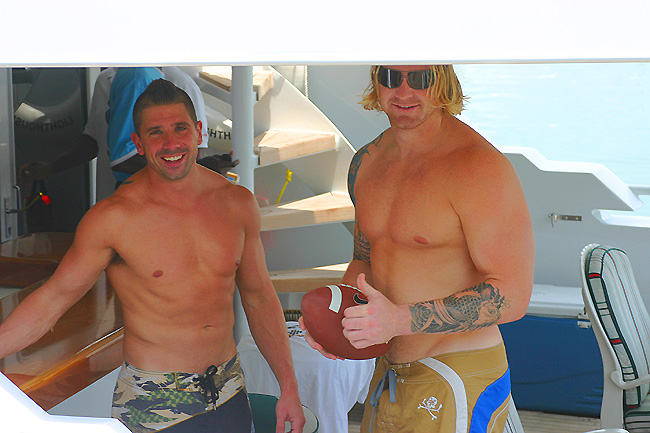The image shows two shirtless young males on a boat, posing and smiling directly at the camera. The young man on the left has short, dark hair styled in a slight mohawk, resembling Aaron Hernandez. He is wearing swim trunks and appears to be in his thirties or forties. The taller man on the right has medium-long blonde hair, is wearing black sunglasses, and also appears to be in his thirties or forties. He is holding a football in his left hand and has a tattoo on his left forearm. His swim trunks are a combination of yellow, white, and blue. Behind them, parts of the boat are visible, including stairs, a cushioned white seat, and a door, with water in the background suggesting they are on a lake or ocean. The weather is sunny, adding to the cheerful atmosphere of the scene.